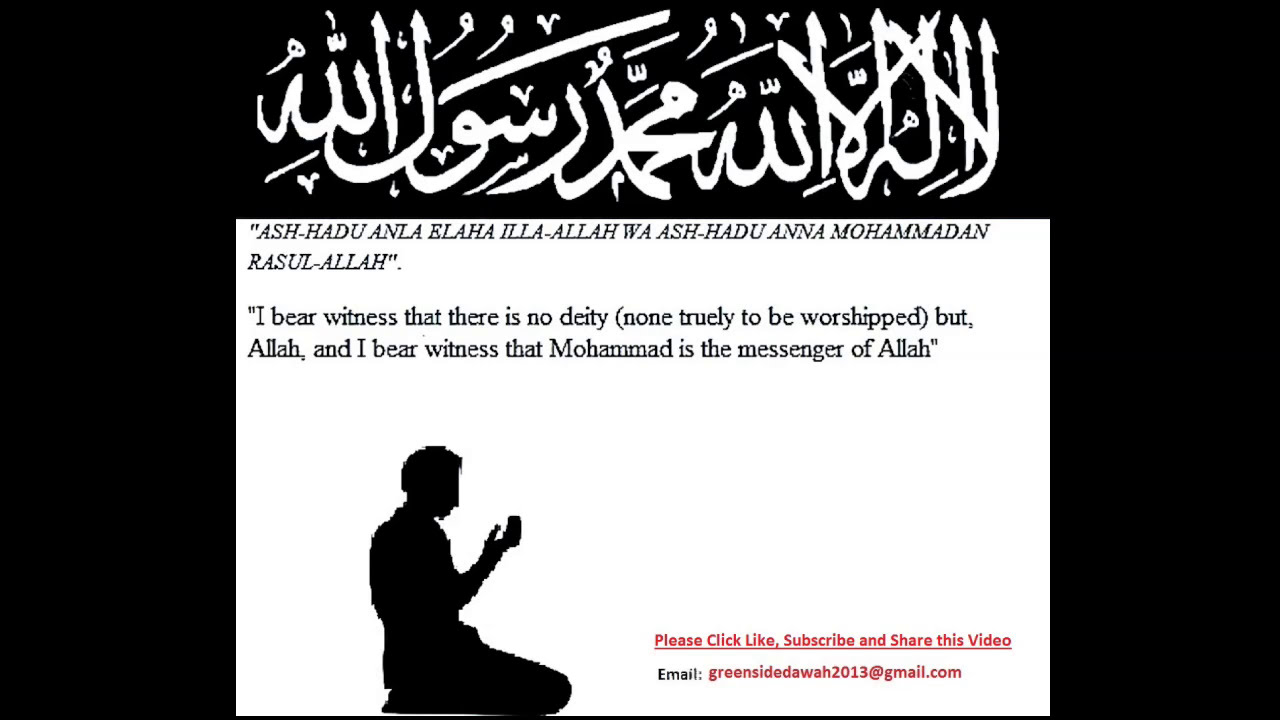The image is a wide rectangular digital artwork or screenshot with a black background. At the top center of the image, there is stylized Arabic text. Below this, stretching down to the bottom, is a large white rectangle. Inside the rectangle, at the top, text appears in all capital English letters that transliterate Arabic words: "M-M-A-D-A-N" on the first line, "R-A-S-U-L" on the second, followed by "A-L-L-A-H" in parentheses. Beneath this, a translation reads, "I bear witness that there is no deity, none truly to be worshipped but Allah, and I bear witness that Muhammad is the messenger of Allah."

The bottom section of the rectangle features text in pink and black. It says, "Please click like, subscribe, and share this video," followed by a black "email;" and in pink, "greensidedawa2013@gmail.com." A black silhouette of a man kneeling with his palms facing upwards, looking at his hands, is also depicted, positioned towards the right of the image.